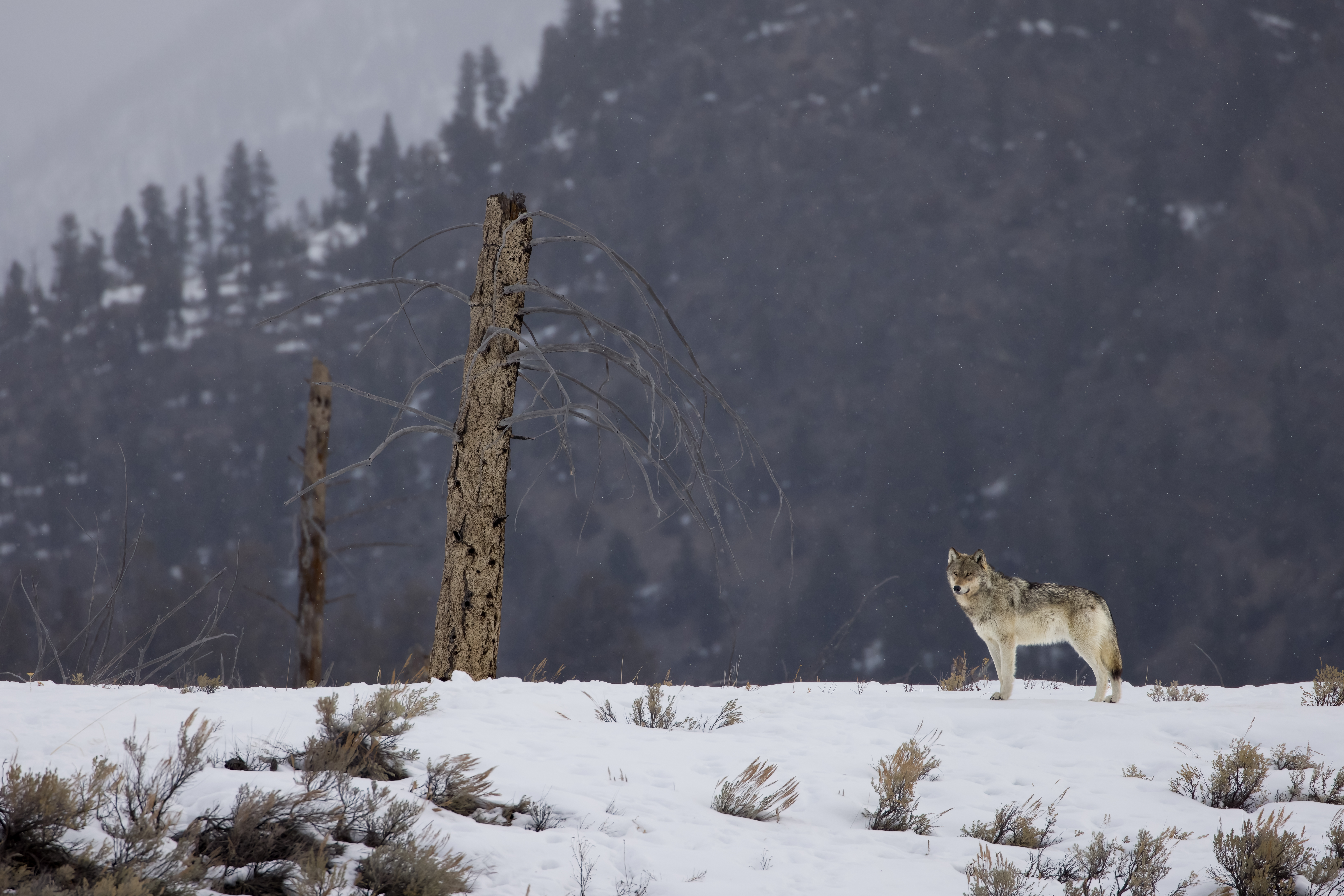In this professionally captured outdoor photograph taken during winter, a lone wolf stands prominently on the right side of the image on snow-covered ground with patches of dry, tan-colored grasses and shrubs protruding through the snow. The wolf, showcasing a mix of black, white, and brown fur on its upper body, and white with tan on its underbelly and legs, gazes towards the camera from a distance. Its distinguished black-tipped tail adds to its striking appearance. On the left side of the image, two tree trunks stand eerily; one, robust yet truncated, with dead twigs branching out, and the other, slimmer and barer. These trunks are devoid of leaves, suggesting the harshness of the environment. The backdrop features a dense forest of coniferous trees, their dark green hues muted by the cloudy or possibly snowy sky. The upper left-hand corner of the image hints at a distant mountain or sky with a medium gray tone, adding depth to this serene and stark winter landscape.